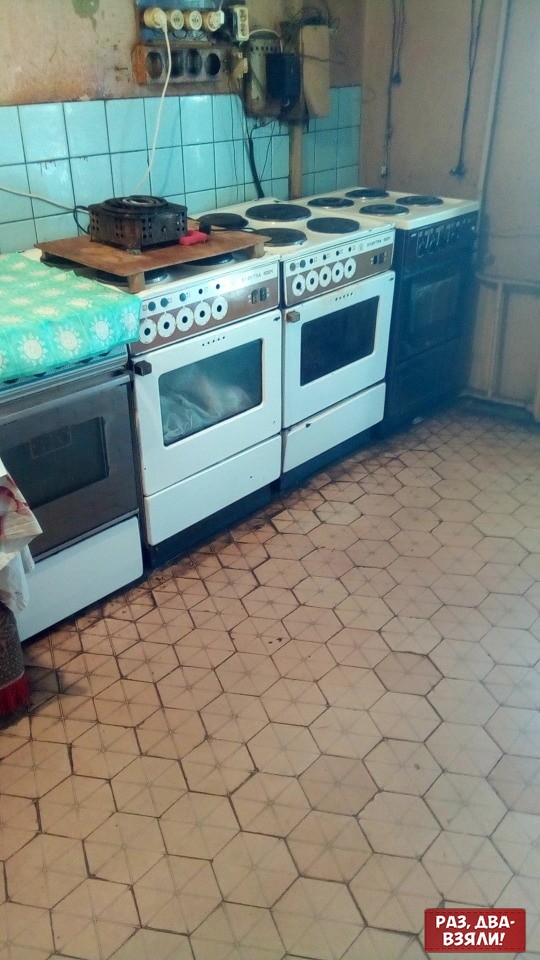The photograph depicts a somewhat dingy, old-fashioned kitchen with four electric stoves and ovens lined up side by side, from left to right. The stoves appear to be predominantly to the left side of the image, with the photo taken at an angle revealing the front of each appliance. The first stove on the left has a black body with a white hob and is partially covered by a blue and white cloth. The two middle stoves are entirely white and the one on the left has a metal plate and a cooking device sitting on the hob, while the one on the right is bare. The final stove on the right side is all black. All stoves are positioned against a wall adorned with green and light blue tiles, stretching from the stovetops to high up the wall. Directly below each stove, the linoleum floor, which features a tan hexagonal pattern, shows marks of dirt. Additionally, a large electrical outlet panel is visible behind the stoves, serving as a connection point for all the appliances.